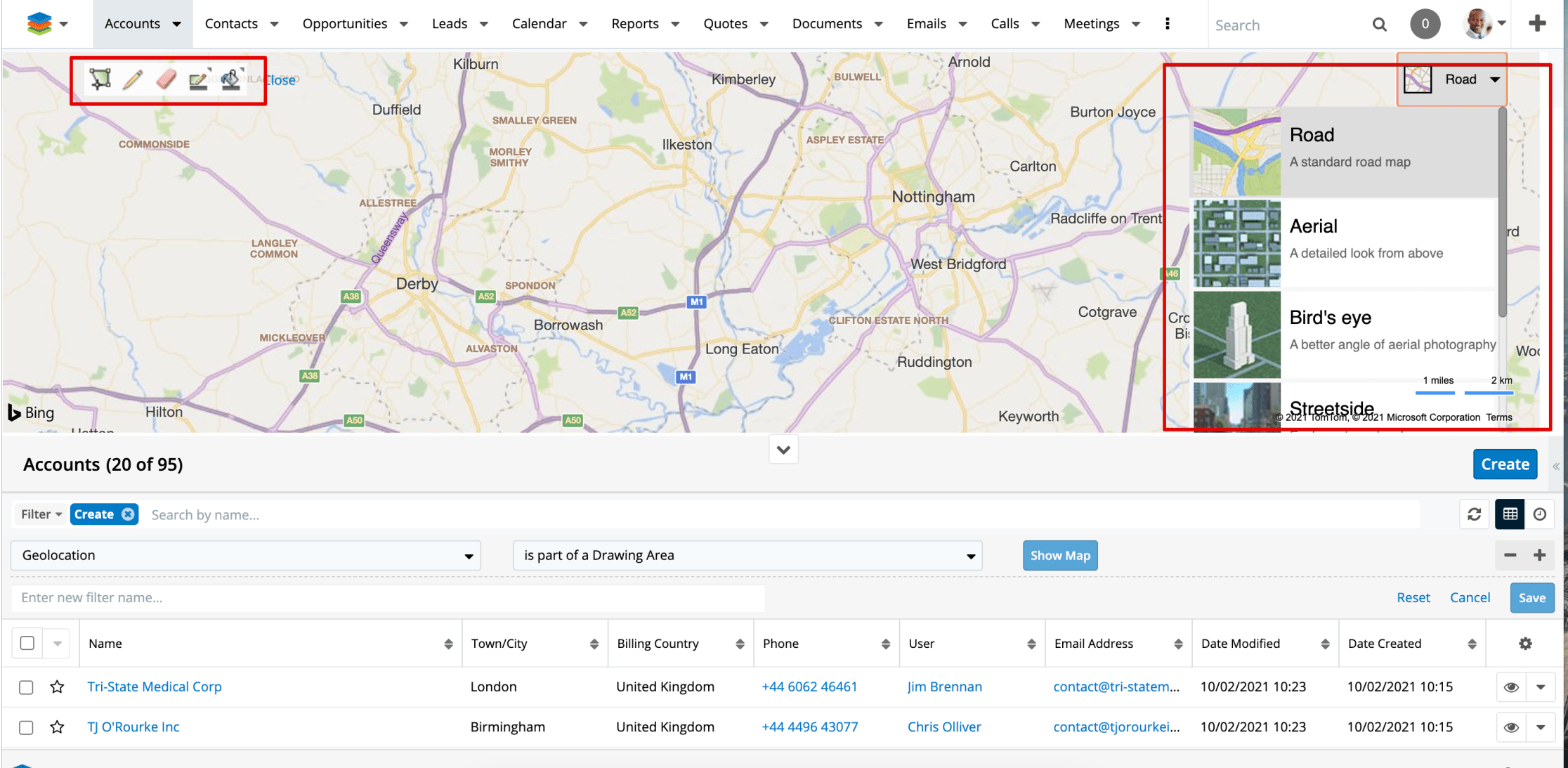In this detailed image, the top section prominently features a map showcasing multiple locations, including Hubern, Duffield, Kimberly, Burwell, Aspley Estates, Allestry, Langley Common, Commonside, Mikulova, Hilton, Derby, and Burwash. Below the map, a user-friendly dashboard is displayed with various dropdown menus for accounts, contacts, opportunities, leads, calendar, reports, quotes, documents, emails, calls, and meetings.

To the right of these menus, there is a search bar accompanied by a search field, enabling efficient data retrieval. The user's profile photo is also visible within this interface. Specific details displayed in the interface include geolocation information, the name "Tri-State Medical Corp," located in London, United Kingdom, along with associated email addresses, dates modified, and dates created. This comprehensive view offers a detailed overview of various business components and their respective statuses.